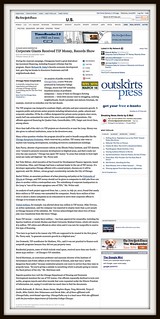The image depicts a highly blurred screenshot of what appears to be a website named "Outskirts Press." The site's design resembles that of a local newspaper or journal, featuring a two-column format. The left column is densely packed with text, likely containing a significant news article or informative content. In contrast, the right column includes advertisements and navigational links to other parts of the website. 

At the top center of the right-hand column, the website's name "Outskirts Press" is prominently displayed, with "Outskirts" written in dark blue and "Press" in light blue. The overall color scheme includes a white background with predominantly black text, accented by blue hyperlinks.

The image is framed by two borders: an inner border in light beige or tan, and an outer black border, giving it the appearance of a framed picture. Due to the extreme blurriness, the only legible text is "Outskirts Press," and the details of the content within the website remain indistinguishable.